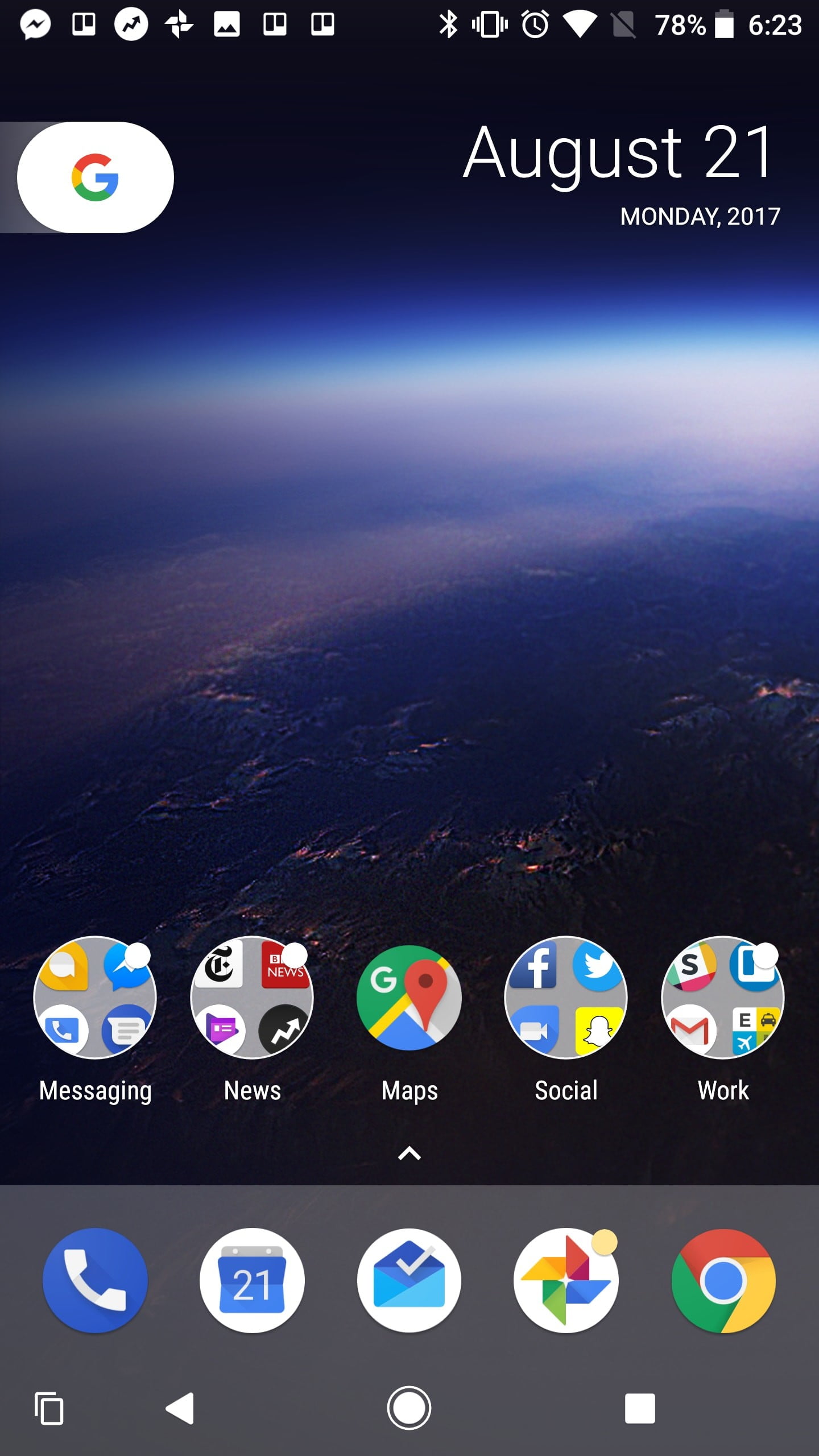This is a detailed screenshot of a phone's screen saver. The background is a serene night sky, transitioning into foggy clouds, and further down into mountainous terrain at the bottom. Spanning the top of the screen is a black band running horizontally from left to right. In the upper left corner, there is a series of icons: a speech bubble containing a small message, a square divided by two rectangles, a circle with a squiggly line, a pinwheel icon, and a picture icon followed by two additional squares each with small rectangles inside. 

To the right of these, there are several status indicators: a Bluetooth icon, a cell phone signal icon, an analog clock, a Wi-Fi signal indicator, a muted speaker icon, a battery percentage reading 78%, and a battery level indicator. The time displayed is 6:23.

Beneath these indicators, towards the left, there is a white oval featuring a multicolored Google 'G', a combination of red, yellow, green, and blue. Adjacent to it, in white text, is the date "August 21, Monday 2017".

Towards the bottom section of the screen, there are two rows of icons. The top row consists of: Messaging, News, Maps, Social, and Work icons. The bottom row features: a phone handset, a calendar icon marked with "21", an envelope, a pinwheel, and the Google Chrome icon.